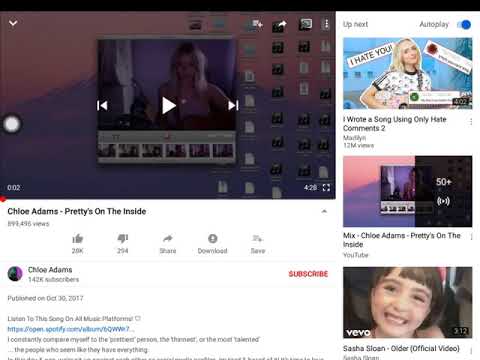Screenshot of a desktop with a web player open in the foreground, numerous document icons in the background. The web player occupies a small square space and displays a performance by a blonde artist named Chloe Adams. The player interface includes play, rewind, and forward buttons. Below the player, text reads "Chloe Adams, Pretty on the Inside" with a view count of approximately 899,495. Additional interface elements include thumbs up, thumbs down, share, download, and save buttons. The description highlights Chloe Adams having 142,000 subscribers with a prominent red subscribe button nearby. On the right side of the screen, there's an autoplay menu featuring three other tracks, including one by Chloe Adams and others by different artists from platforms like YouTube and Vevo.